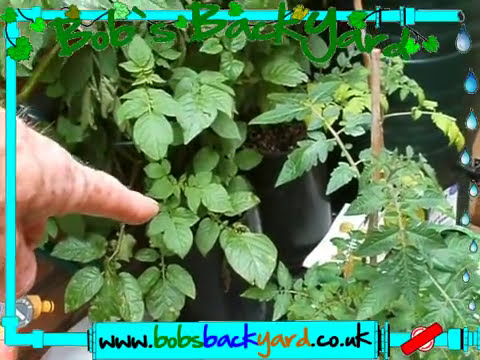The image depicts a detailed gardening scene prominently featuring green tomato vines without visible tomatoes. In the foreground, a person's hand is shown in the lower left-hand corner, with the index finger pointing towards the vines, adding a personal touch to the scene. The top of the image displays the text "Bob's Backyard" in green font, framed by a blue border that runs around the entire edge of the picture. On the bottom, the website "www.bobsbackyard.co.uk" is displayed, with "www" in black, "Bob's" in green, "Back" in blue, "Yard" in orange, and "co.uk" in black.

On the right-hand side, an open faucet is dripping water onto the tomato plants, with visible drops cascading down. There is also a red valve on the lower right-hand corner of the blue-bordered pipe. The plants are situated in black planters with visible soil, and smaller green leaves surround the tomato vines. The meticulous layout and elements suggest it could be an instructional video or a visual guide related to gardening, highlighting the care and attention Bob dedicates to his backyard plants.